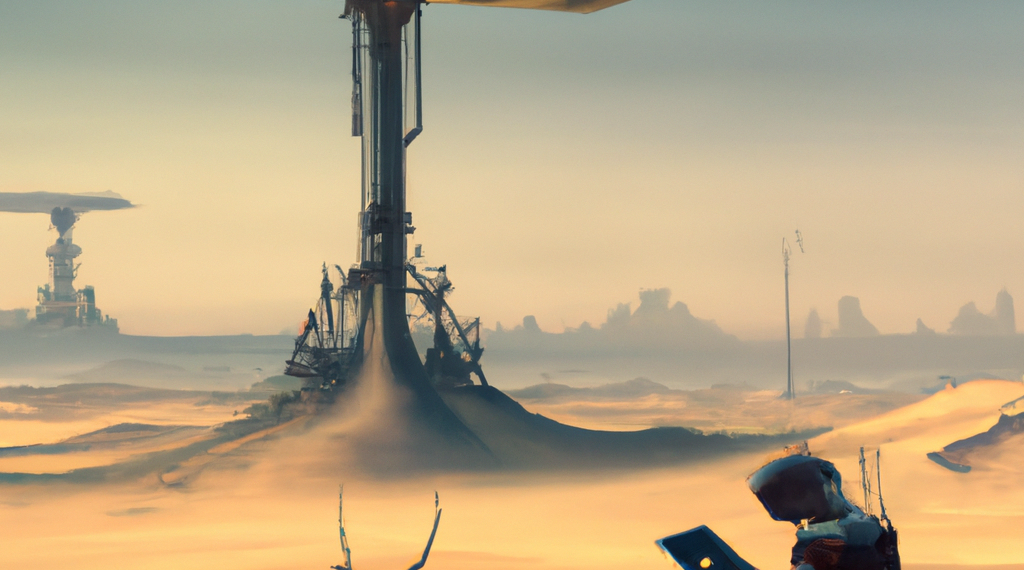The wide rectangular digital artwork illustrates a sci-fi scene set in a desolate and uninhabited landscape, reminiscent of a video game environment. The foreground features light yellow and dark gray clouds that create a stark contrast at the bottom of the image. Just to the left of the center, a tall gray apparatus with a narrower top rises out of the dark gray clouds, suggesting an antenna or tower. In the distance, to the left at the horizon line, another similar tall gray apparatus is visible between two horizontal dark gray clouds, adding depth to the scene.

The sky above fades from a light bluish gray at the top to a light yellowish gray near the horizon, evoking a twilight atmosphere. The terrain below, resembling a desert with dunes, transitions from piles of sand encircling the towers to a distant horizon line with outlines of more solid structures. 

In the bottom right corner, a person wearing a gray, metallic helmeted suit is depicted looking down at a screen, lending an impression of technology and exploration. Antennae emerging from the bottom of the picture further enhance the otherworldly feel, giving a sense that this scene might be set on another planet.